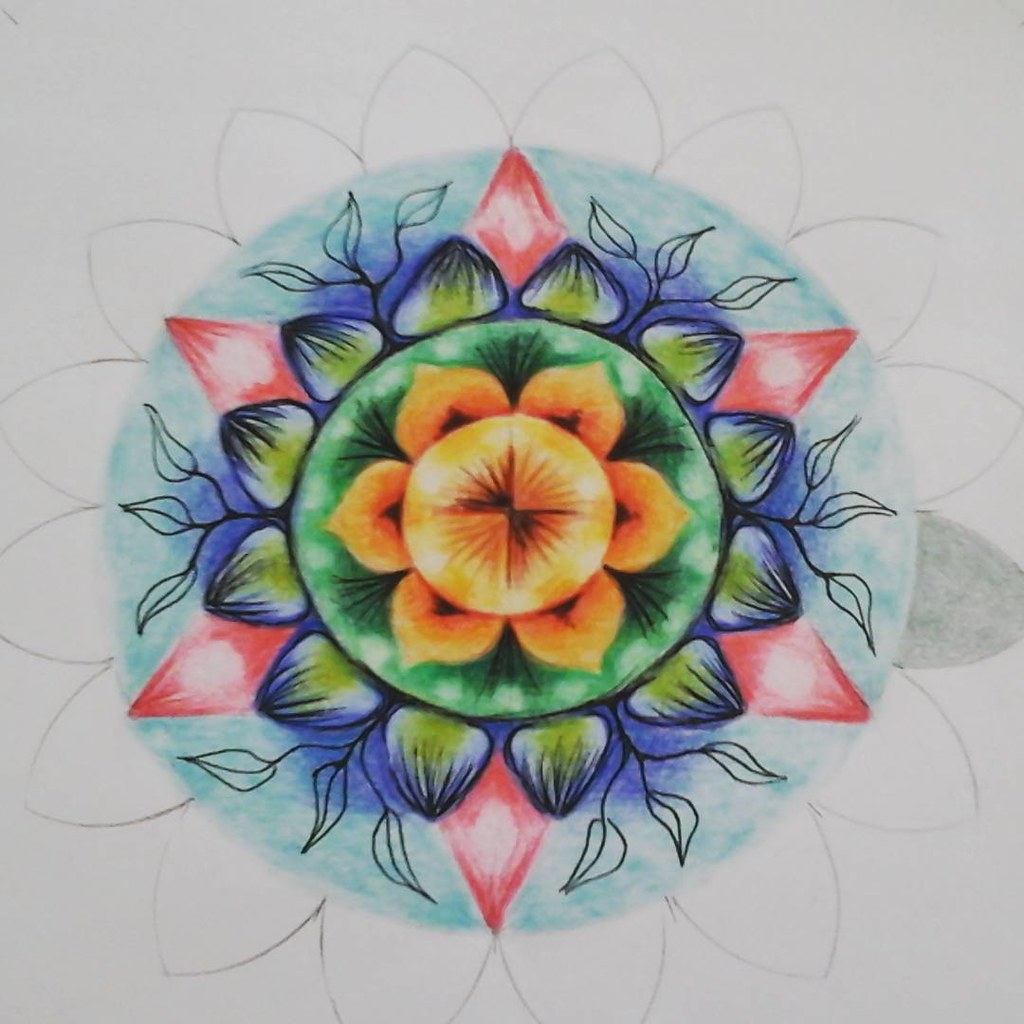The image on a white background depicts a highly detailed, surreal, and symmetrical floral design that appears to be AI-generated. At the heart of this intricate composition is a large yellow flower with six petals, set within a yellowish-orange, hourglass-shaped core. Surrounding this central flower is a green circular band adorned with small white dots. Encompassing this green band is a blue ring resembling a series of guitar pick-shaped petals, each outlined in dark blue with green interiors.

Moving outward, the next layer is a lighter blue circle featuring red crystal diamond shapes positioned at uniform intervals, analogous to clock face positions: at 12, 2, 4, 6, 8, and 10 o'clock. Beyond this is a pencil-drawn ring of uncolored petals with one shaded in grey, enhancing the layered and hand-sketched aesthetic. The entire arrangement has an almost brooch-like appearance, blending vibrant colors with meticulous design, completing a multi-floral, concentric circular pattern that appears both organic and digitally refined.